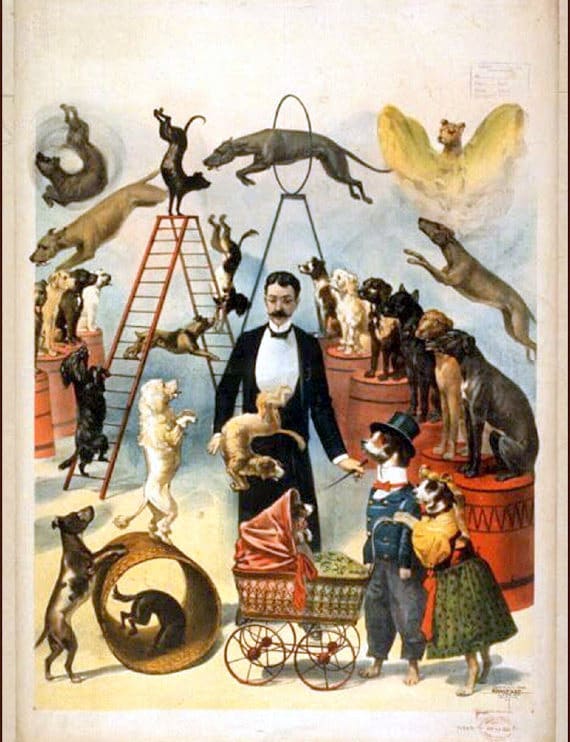This vintage circus poster features a central gentleman with a dark black mustache, dark 1800s-era hair, and a black tuxedo with a white shirt and black bow tie, orchestrating a lively dog performance. Around him, a variety of dogs exhibit impressive feats. In the bottom left corner, a small dog pushes an open barrel containing another dog, while a white, poodle-like dog balances on its hind legs on top. To the right, two dogs dressed as a man and woman—a Saint Bernard type in a black top hat and a smaller dog in a dark green dress—push a pram with an orange top, wheeling another small dog inside. In front of the man, a dog executes a somersault. Nearby, several dogs, resembling whippets or greyhounds, sit on or leap behind barrels. High in the background, a Great Dane jumps through a hoop attached to a ladder, while another dog performs a handstand atop an orange-ish ladder. This dynamic illustration captures the essence of an old-time dog circus, with the ringleader commanding a myriad of canine tricks and stunts.